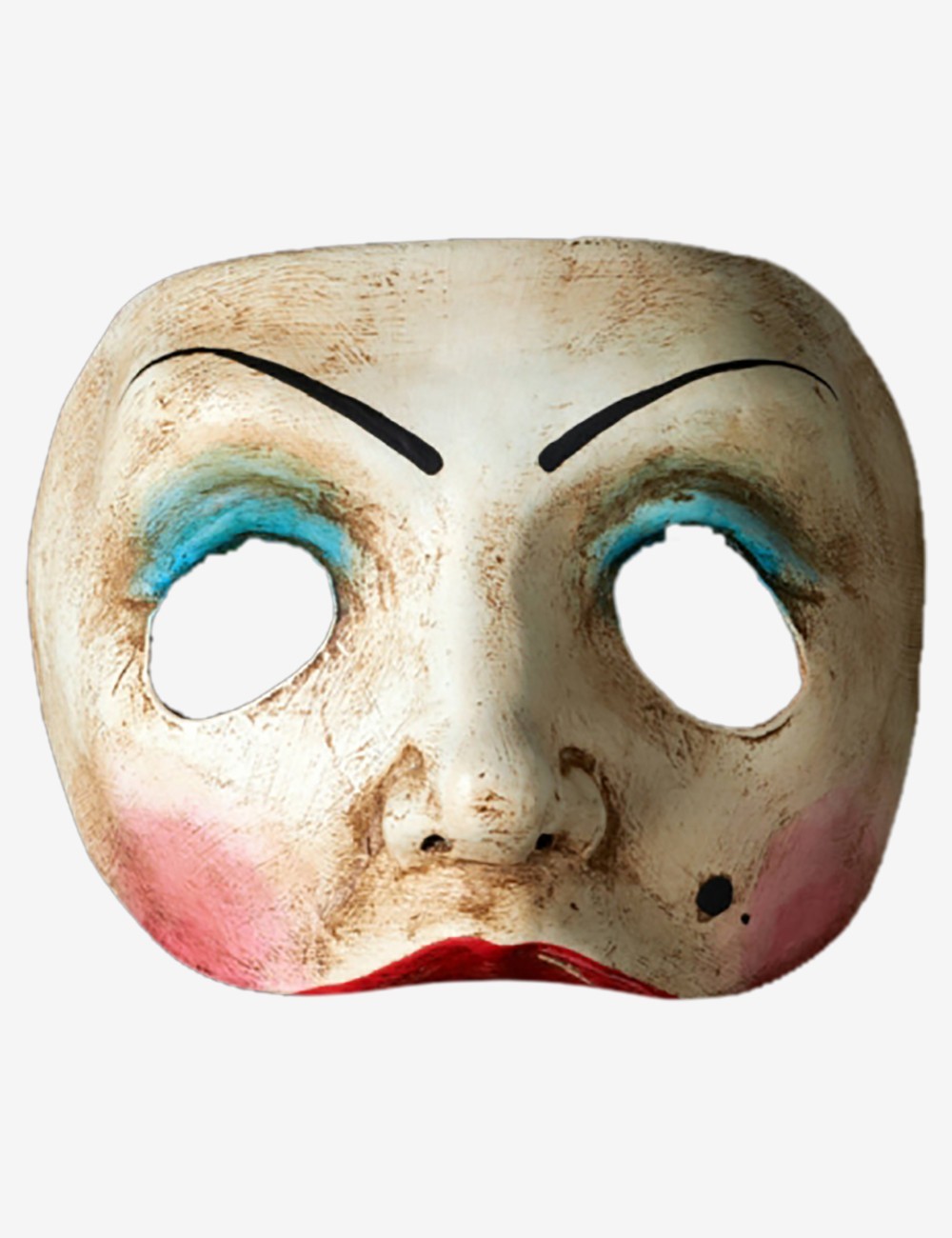The image features a detailed, vintage mask set against a plain white background, which underscores its antiquated and worn appearance. The mask, evocative of something one might wear in New Orleans, is cut off just below the upper lip, revealing a vividly painted deep red lipstick on the lips. The mask itself is predominantly off-white or ivory, though its surface is marred by dirty brown streaks, giving it an aged look. The eye holes are framed by bright, sky-blue eyeshadow, and the mask features very thin, sharply drawn black eyebrows above these eyes. Highlighting its rosy cheeks, there is a notable pink-red blush. A distinctive mole is located above the upper lip on the right side, emphasizing the mask's detailed representation of a woman's face. This highly descriptive mask captures elements of both elegance and wear, presenting a striking and evocative image.